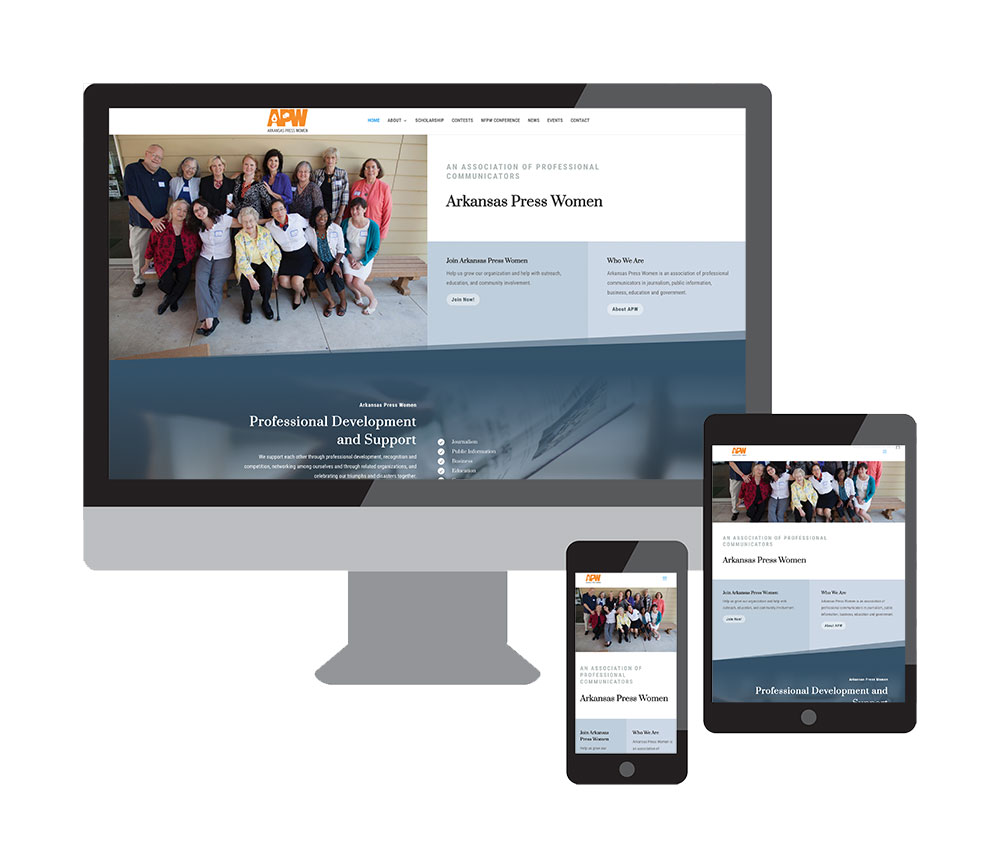The image is a digital illustration showcasing how the Arkansas Press Women website appears on various devices: an iMac, a tablet, and a smartphone. Each device screen displays the homepage of the website, accurately representing its responsive design across different platforms. The website features a banner that reads "Arkansas Press Women: An Association of Professional Communicators." On the left side of the homepage, there is a prominent photo of a large group of individuals, predominantly women, either seated on a bench or standing behind it, leaning against a beige wall. The homepage also includes several columns with detailed sections: 'Join Us', 'Who We Are', and 'Professional Development and Support'. Each section offers further insights, including bullet points under 'Professional Development and Support', outlining various opportunities and resources provided by the association.